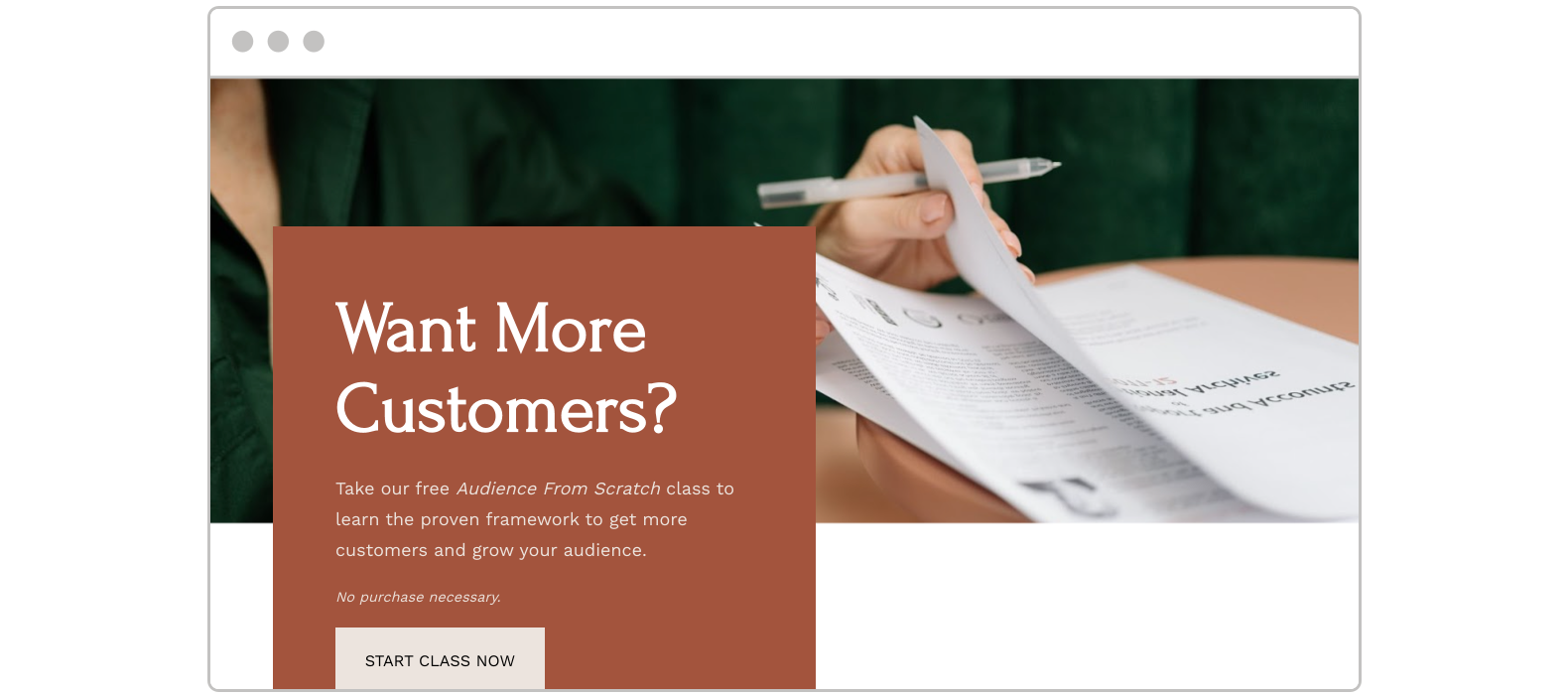The image appears to be a mock-up of a website displayed on a Mac browser. At the top, the browser window is visible with three dots on the left, indicative of macOS. The main section of the mock-up features a hero image of a woman dressed in a green silk shirt sitting at a wooden table. She is holding a pen and flipping through some papers. In the background, green curtains are visible, adding a cohesive color element to the image.

On the left half of the image, there is a brown overlay that covers most of the top portion and extends to a white area below. Superimposed on this overlay is black text that reads: "Want more customers? Why take a free audience from scratch class to learn the proven famous framework to get more customers and grow your audience. No purchase necessary." Below this text is a white button with the phrase "START CLASS NOW" in capital letters.

The entire mock-up is framed with a thin gray outline, giving it a neat and contained appearance. Overall, the design is simple and appears to be an unfinished sign-up page for an unspecified company, as no branding information is present.